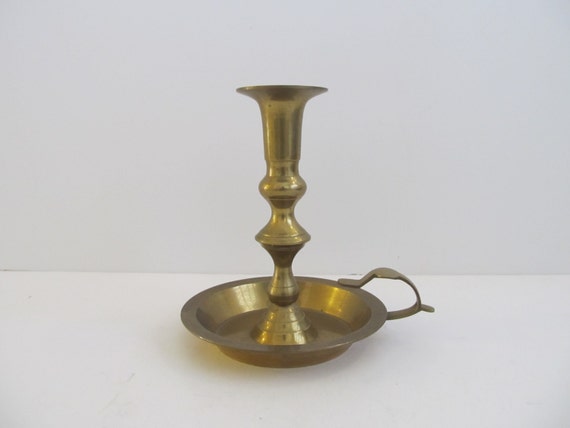The image showcases a tarnished gold, metallic candle holder set against a neutral white surface, likely to highlight its features. The structure comprises a shallow, circular bronze dish positioned on a white base with a ring handle on the right side. Rising from the center of this dish is a tall, vase-like metallic tower with distinct segments; it broadens and narrows in sections before flaring out at the top like a funnel. The topmost part of the tower features three wing-shaped elements, and the base transitions into a triangular shape. The backdrop consists of a white wall, emphasizing the candle holder’s intricate design and antique allure.